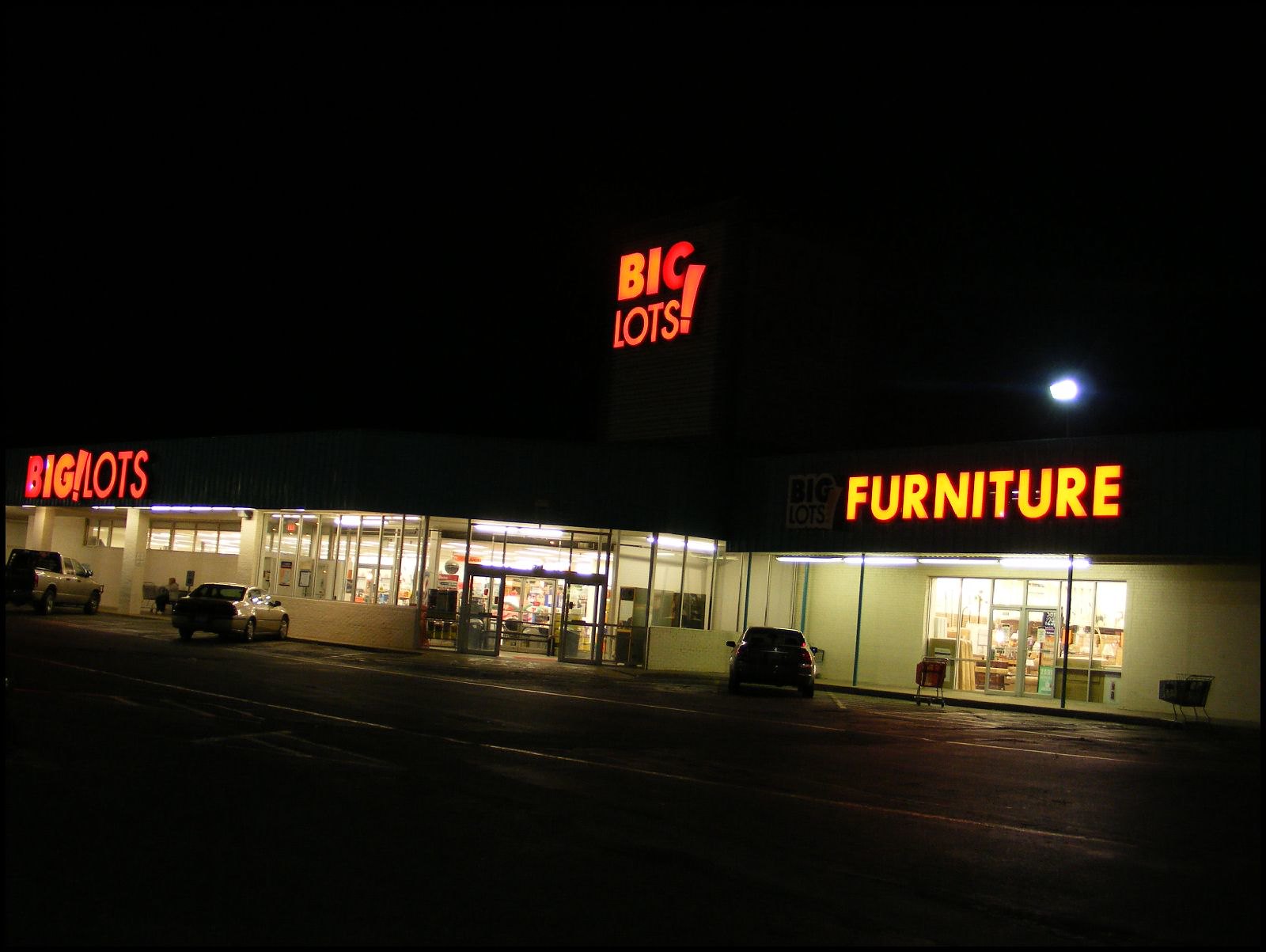The image depicts a Big Lots Furniture Store taken at night, possibly from the parking lot, though it's difficult to discern due to the darkness. The most striking feature is the Big Lots sign with an exclamation point, illuminated in a red-orange color, prominently displayed above the building. The storefront itself reveals "Big Lots" on the left side and "Furniture" on the right, both brightly lit. Despite the nighttime setting, the surrounding area is dimly lit by a bright spotlight above the "Furniture" sign. No stars or moon are visible in the dark sky. In front of the store, there are two cars and a truck parked, alongside three grocery carts that have been left outside. The building's cream color contrasts with the glow from inside the store, visible through the glass windows, adding to the scene's overall detail and ambiance.